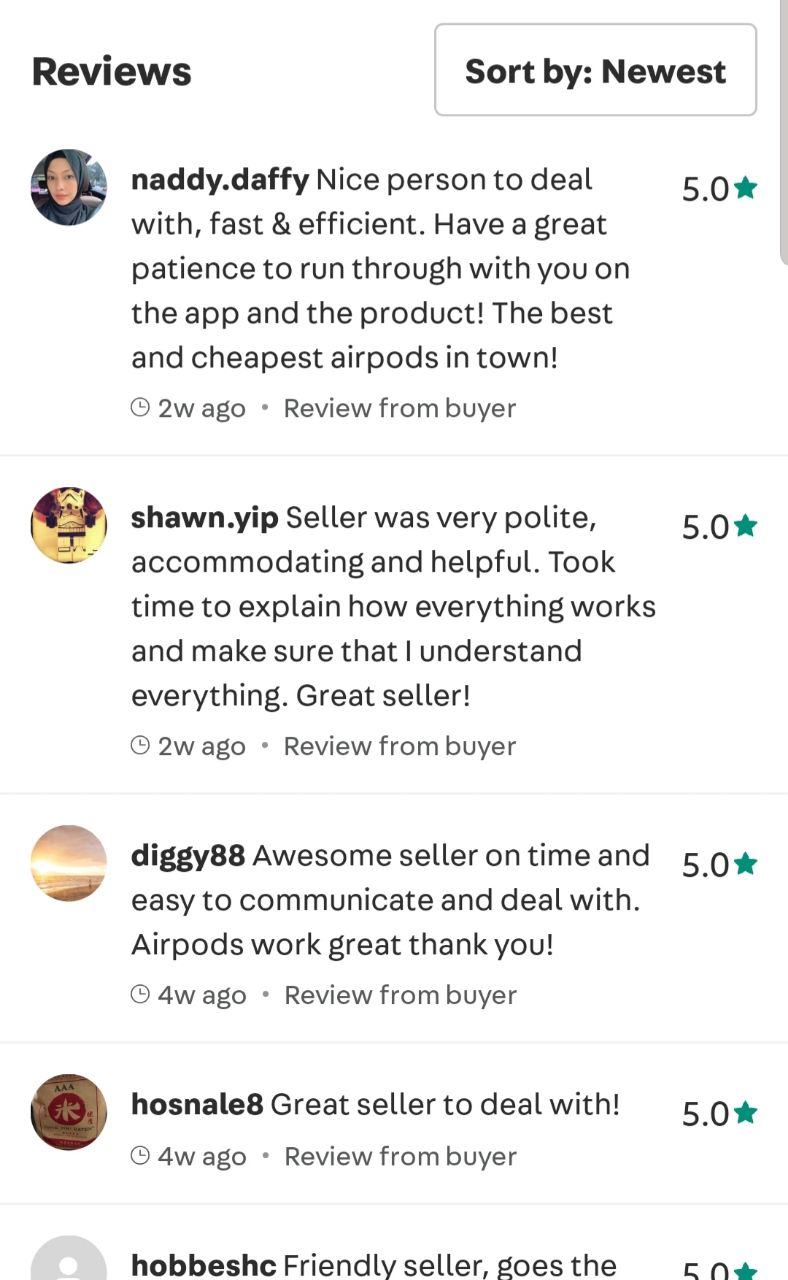The image features a white background with a header at the top labeled "Reviews." Below the header, there's a small box labeled "Sort by Newest." On the right side of the image, a faint gray line is partially visible. On the left side, a small circle contains the profile picture of a user named Natty.Daffy. The review by Natty.Daffy reads: 

"Nice person to deal with, fast and efficient. Has great patience to run through the app and product with you. The best and cheapest AirPods in town." 

Next to this review, there's a small clock icon indicating the review was posted two weeks ago, a label "Review from Buyer," and a rating of 5.0 stars.

Below this, another review by Sean.Yip states: 

"Seller was very polite, accommodating, and helpful. Took time to explain how everything works and made sure that I understood everything. Great seller."

This review also has a clock icon indicating it was posted two weeks ago, a "Review from Buyer" label, and a 5.0-star rating highlighted in green.

The third review is from Diggy88, who describes:

"Awesome seller, on time, and easy to communicate with. AirPods work great. Thank you."

This review includes a clock icon showing it was posted four weeks ago, a "Review from Buyer" label, and a rating of 5.0 stars.

Further down, a user named HoseNail8 simply reviews:

"Great seller to deal with."

This is also marked with a clock icon, indicating it was posted four weeks ago, a "Review from Buyer" label, and a 5.0-star rating.

Finally, there's a brief review from Hobbish stating:

"Friendly seller," accompanied by a 5.0-star rating.